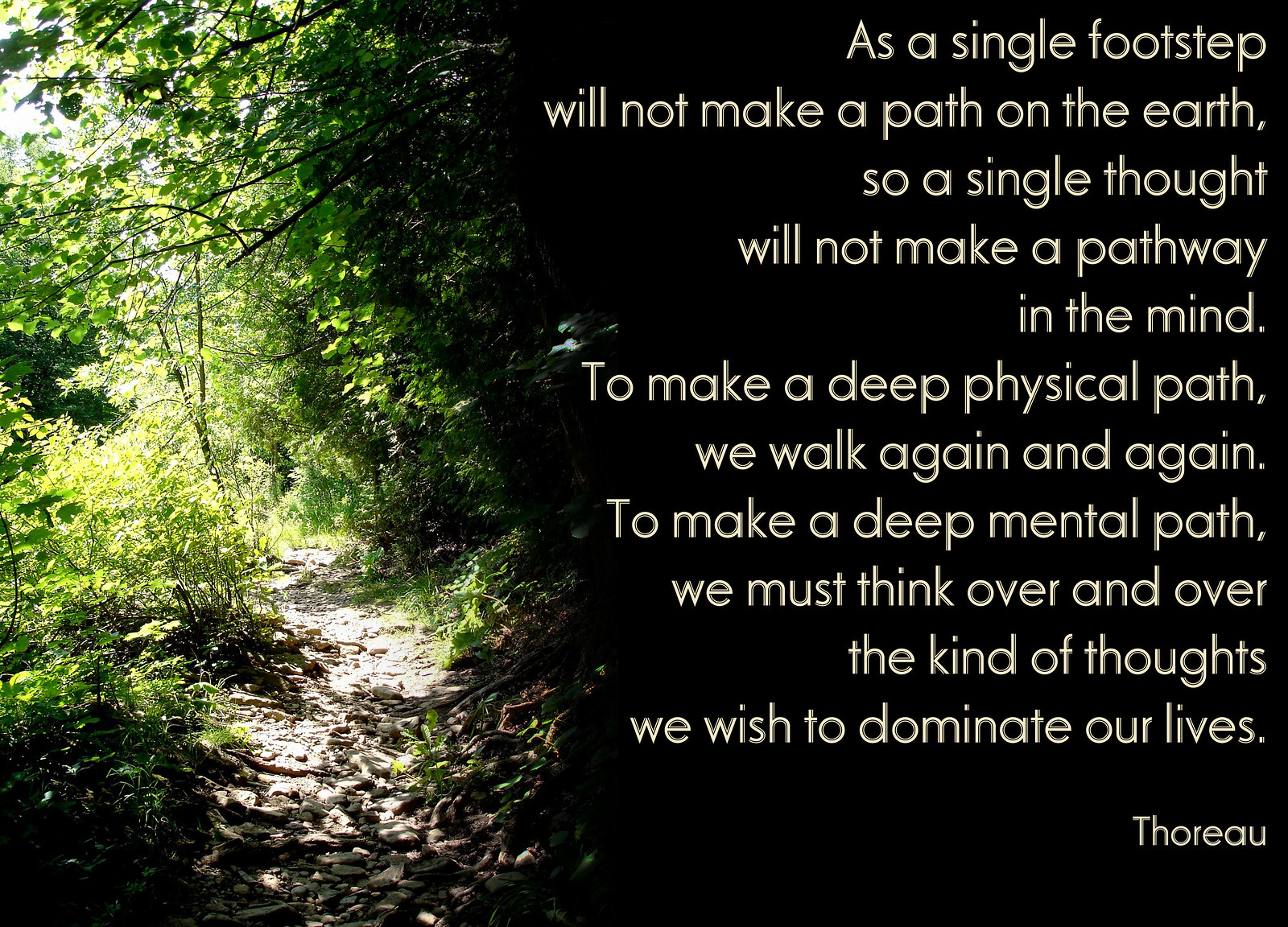The image features an inspirational quote by Thoreau, prominently displayed on the right side in white letters against a black background. The quote reads: "As a single footstep will not make a path on the earth, so a single thought will not make a pathway in the mind. To make a deep physical path, we walk again and again. To make a deep mental path, we must think over and over the kind of thoughts we wish to dominate our lives." Below the quote, the author's name, Thoreau, appears. The left side of the image depicts a serene forest scene with a trail lined with rocks, tree roots, and dense greenery. Overhanging trees and abundant vegetation frame the path, while sunlight filters through, illuminating parts of the trail. At the upper left, a glimpse of the sky adds further depth to the picturesque woodland setting.